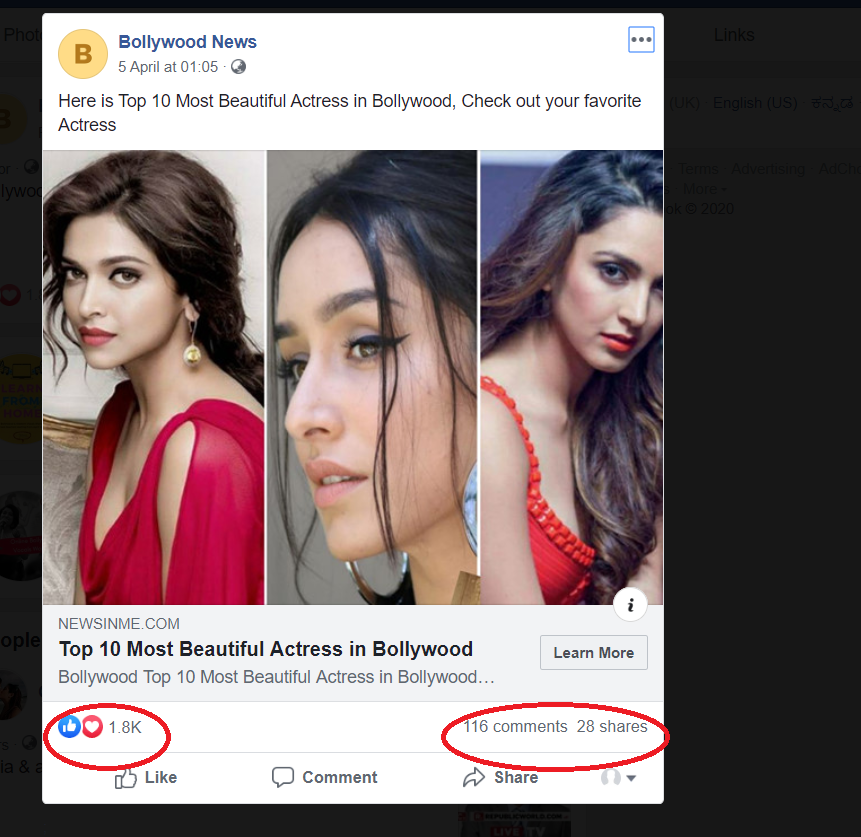The image is a screenshot capturing various elements, with particular emphasis on two red-circled areas. The screenshot appears to be from a webpage, specifically a piece of content titled "Bollywood News," dated April 5th at 1:05. The main headline reads, "Top 10 Most Beautiful Actresses in Bollywood. Check out your favorite actress."

At the top, three actresses with dark hair are featured prominently in a collage. The actress on the left is in a reddish outfit with billowy sleeves, and she is looking towards the camera while her body is angled to the left. In the center, a close-up shot highlights an actress looking to the left, focusing mainly on her face. The actress on the right is dressed in a tight, almost halter-style red top, with her body facing right but her gaze directed towards the camera.

In the middle of the image, there are two significant red circles. The first red circle encompasses a blue thumbs-up icon next to a number, "1.8k," signifying 1.8 thousand likes. The second red circle surrounds a heart icon indicating 116 comments and 28 shares, though the highlighted numbers don't seem proportionate, possibly suggesting some discrepancies.

Underneath, the website's name, "newsinme.com," repeats the headline "Top 10 Most Beautiful Actresses in Bollywood." The call-to-action "Learn More" is visible against a white background, while other details are obscured and grayed out, making them unreadable. 

Overall, the emphasis seems to be on these interactions and the prominence of the article's headline and content.